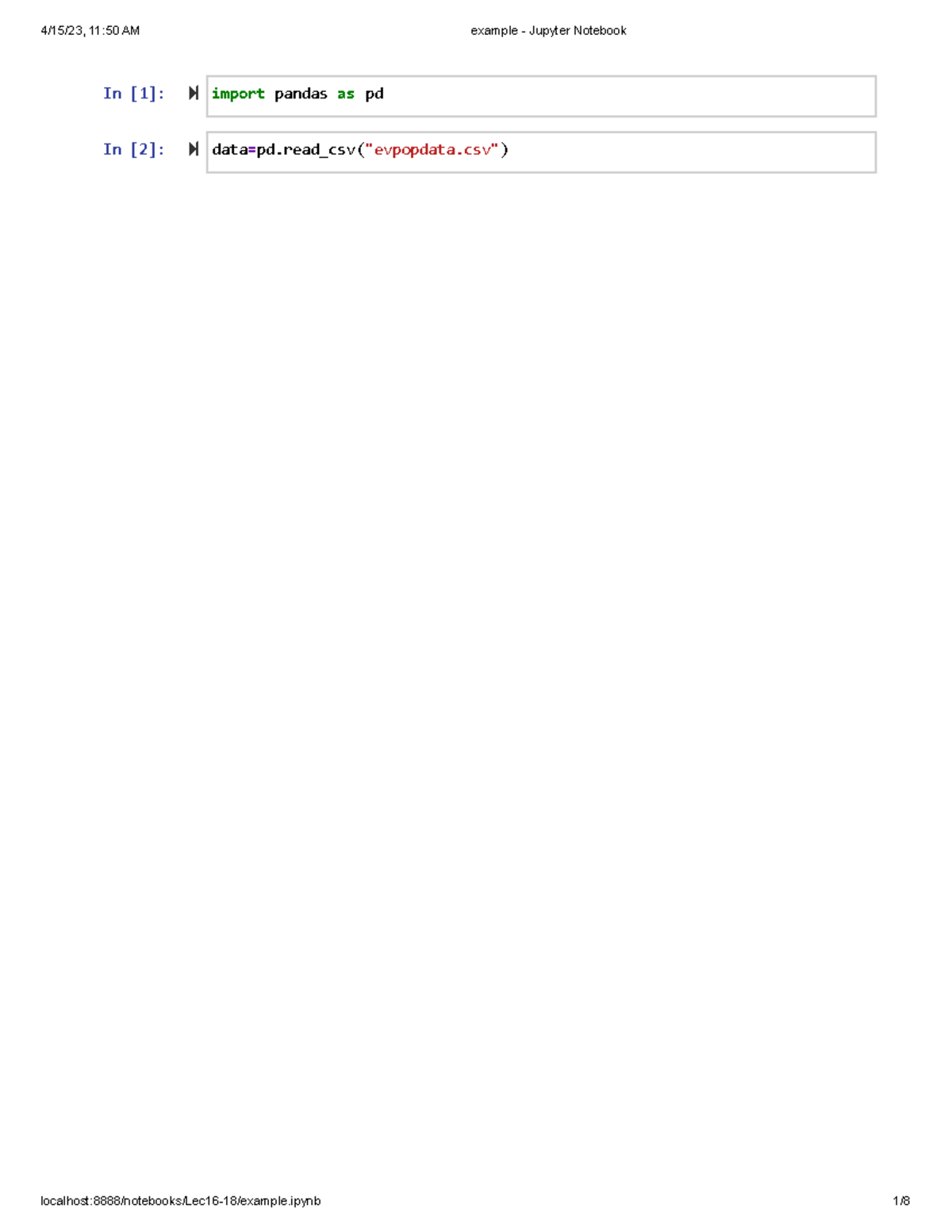**Detailed Caption:**

The image is a screenshot of a Jupyter Notebook interface being accessed through a local server. At the bottom of the page, the footer displays the URL as "localhost:8888/notebook/LLC16-18/example.ipynb," with the page indicator "1/8" positioned to the far right. The header at the top left features the date and time as "4-15-23 at 11:50 a.m." along with the notebook's name "Example-Jupyter Notebook."

Below the header, the notebook interface contains two input cells. Each cell is identified by its respective execution count: the first cell is labeled "In [1]:" in blue text, and the second is labeled "In [2]:" in blue text. Both cells have a right-facing arrow with a vertical line to the left, indicating the input prompt.

In the first cell, the code in green reads `import pandas as pd`, where 'pandas' and 'as' are highlighted in black, and 'pd' is highlighted in green. The second cell contains the code `data = pd.read_csv("EPOPDATA.CSV")`, with the word 'data' in black, the equal sign in purple, and the function `pd.read_csv` in black, followed by the file name "EPOPDATA.CSV" in red, enclosed within black brackets and quotes.

The vast majority of the page, approximately 85% to 90%, consists of white space, making the content within the interface appear notably sparse.